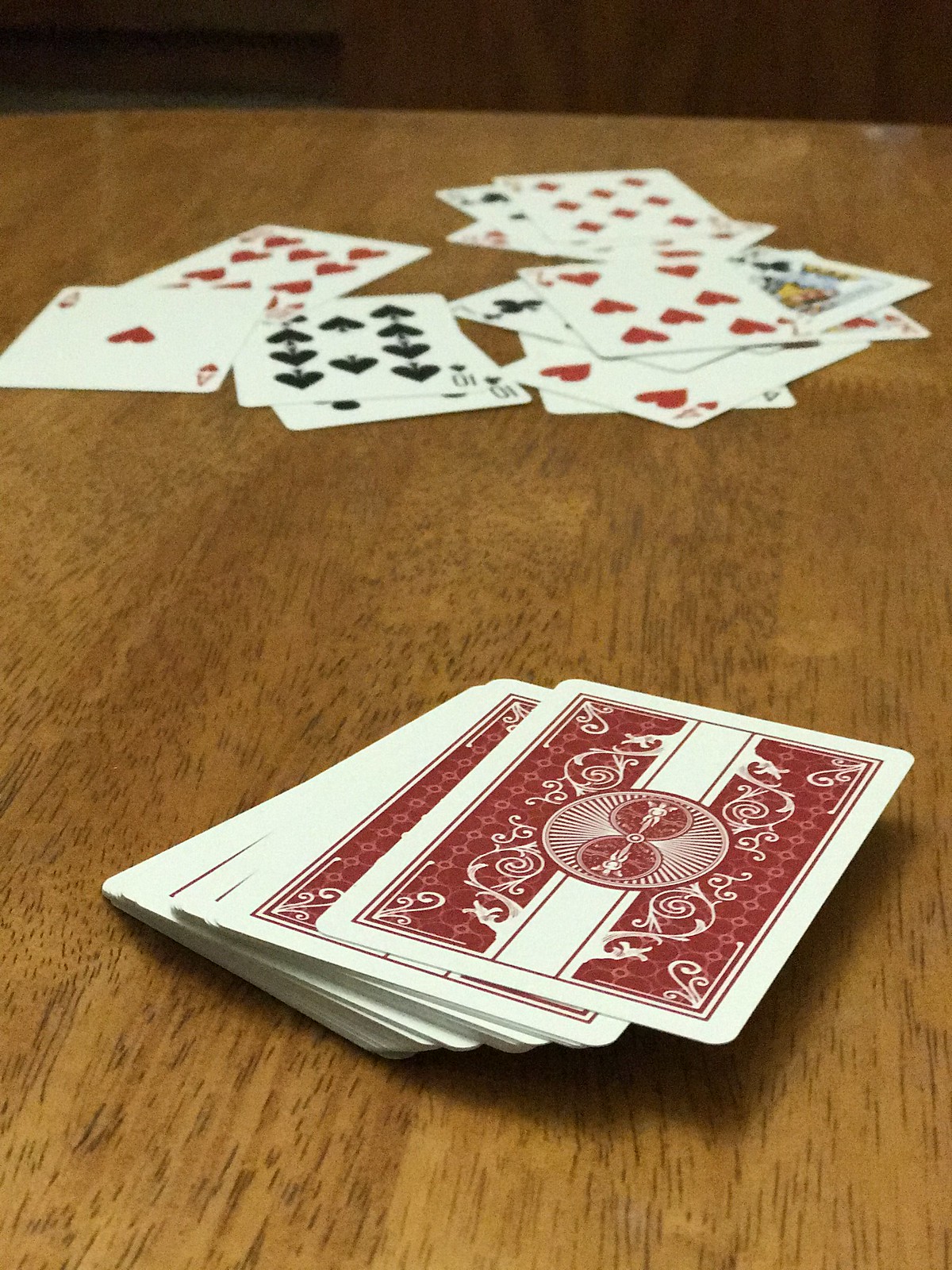In this richly detailed image, a zoomed-in view showcases a wooden table with an intricate pattern of darker wood grains creating swishes and swirls across its brown surface. The table serves as the background for a scattered array of playing cards that appear both in orderly stacks and in casual disarray. 

In the foreground, a deck of rectangular, thin playing cards is neatly piled up. Prominently displayed at the top of this stack is a striking red card featuring a sophisticated design. The card has a white stripe running vertically down its center, which is overlaid with a red circle. Inside this red circle are two smaller concentric circles, and within them, a subtle and intricate figure that resembles a person. The background of the card features a swirly pattern in the red sections flanking the white stripe, which dominates the majority of the card's face.

Behind this red card, a variety of other cards are spread across the table. Notable among them are a red Ace, a black Ten, and a Four of Hearts, each positioned at different angles, adding to the chaotic yet engaging visual arrangement of the scene. Other cards are partially visible, hinting at their identities but remaining indistinct, thus contributing to the mysterious and dynamic nature of the tableau.